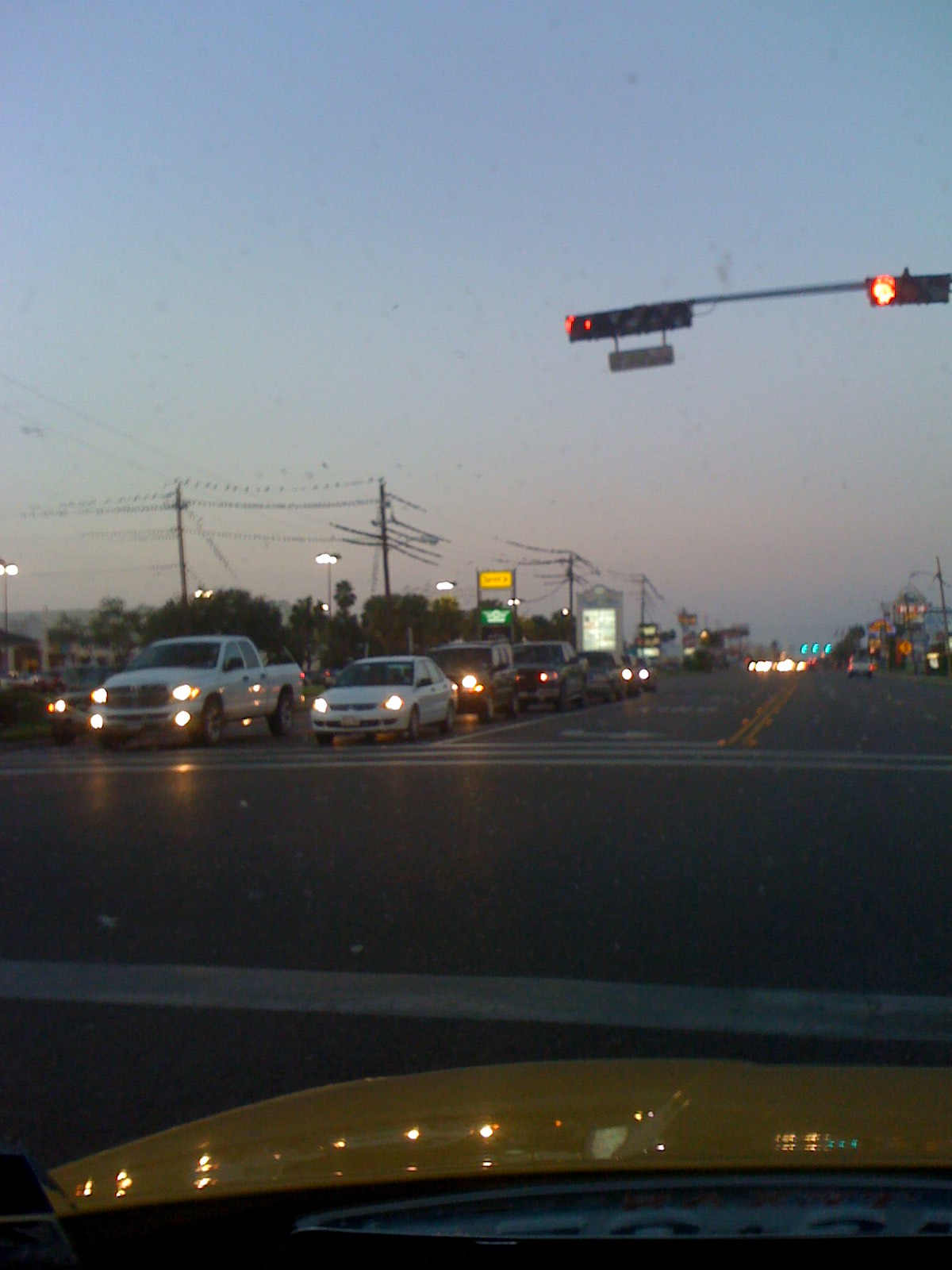This photograph, taken from inside a car with a yellow hood, captures a bustling intersection at dusk or night. The car is stopped at a red light as oncoming traffic, teeming with illuminated headlights, forms a busy queue facing the vehicle from which the picture is taken. Businesses line the sides of the road, their storefronts casting a glow onto the street, while telephone poles and wires crisscross the scene, adding an urban texture. The angle of the shot, whether by the driver or passenger, emphasizes the convergence of vehicles. A yellow traffic sign is visible in the background, along with another street light further ahead, suggesting that the scene could be in the heart of a small town’s main intersection or roadway.